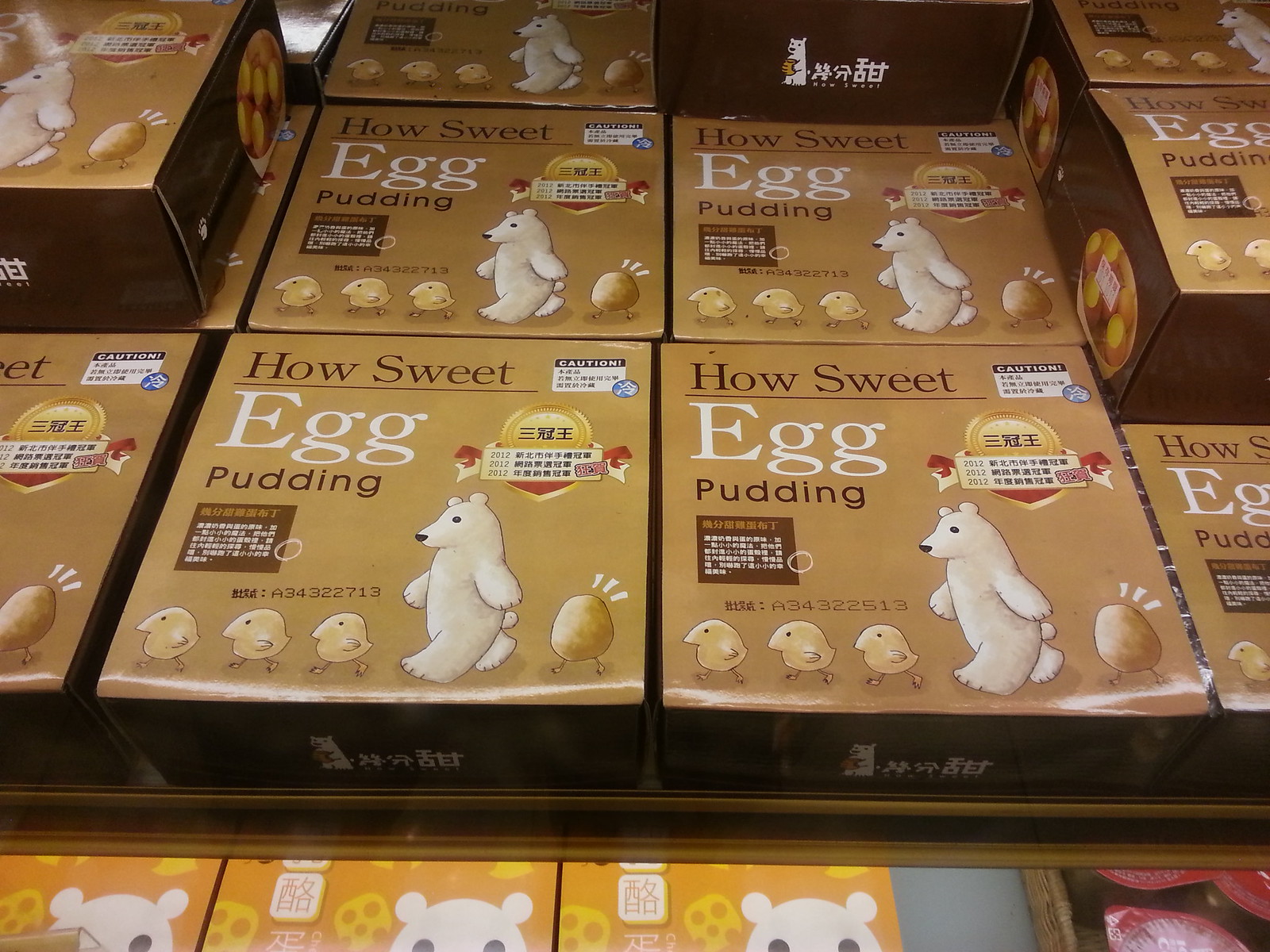The image showcases a store display filled with several caramel-colored rectangular boxes of "How Sweet Egg Pudding.” Each package prominently features a white bear walking towards the left, accompanied by three chicks in front of the bear at the bottom. The design also includes an egg situated behind the bear. In the bottom right corner, there is a small, charming potato figure with legs. The product name, "How Sweet Egg Pudding," is written in bold letters, with the word "egg" in white and the remaining text in black. Additionally, a gold award-like badge with black symbols is displayed on the packaging, along with some non-English text. The top right corner of the package contains a caution label with unreadable words. This visually appealing display shows multiple rows of the product, stacked neatly, while glimpses of an underlying shelf reveal orange packages with the top part of a bear’s head visible.